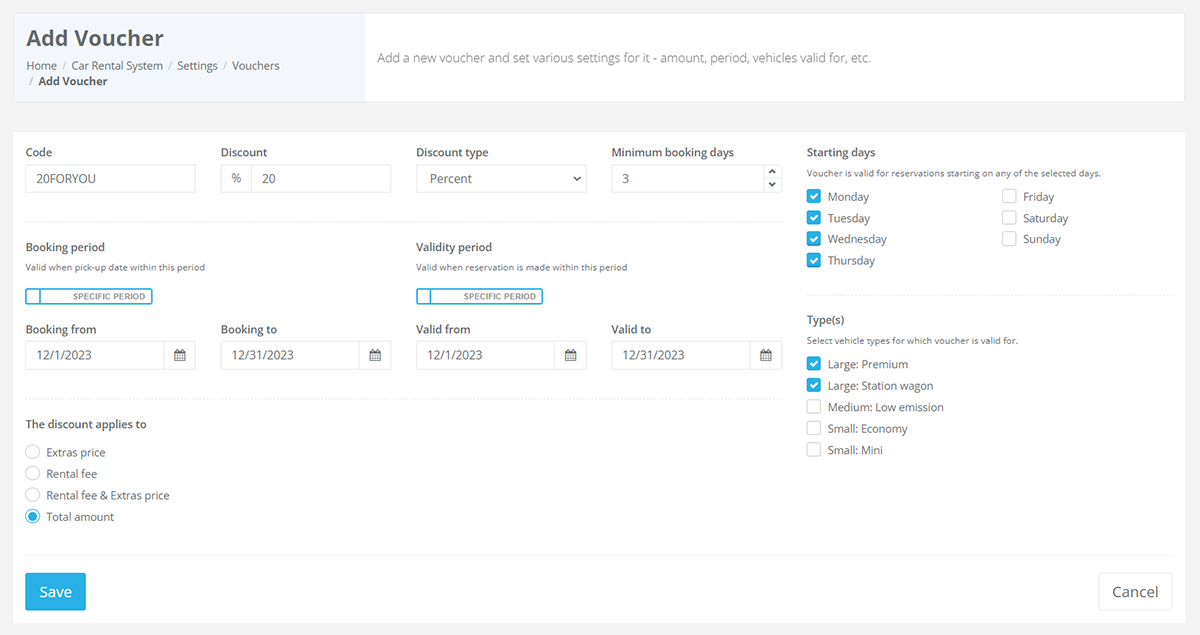This screenshot showcases a section of a web page dedicated to adding a new voucher within a car rental system. The navigation path displayed at the top reads as follows: Home > Car Rental System > Settings > Vouchers > Add Voucher. 

To the right, a header states, "Add a New Voucher and Set Various Settings for It." Detailed input fields and options for configuring the voucher are presented:

- **Code**: 24UFORYOU
- **Discount**: 20%
- **Discount Type**: Percent
- **Minimum Booking Days**: 3 days

Additionally, there are specific settings regarding the validity and applicability of the voucher:

- **Starting Days**: Voucher is applicable for reservations starting on Monday, Tuesday, Wednesday, and Thursday.
- **Booking Period**: Valid for bookings made from December 1, 2023, to December 31, 2023.
- **Validity Period**: The voucher can be used if the reservation is made within the same period, from December 1, 2023, to December 31, 2023.

Furthermore, users can select the vehicle types for which this voucher is valid:
- Large Premium (selected)
- Large Station Wagon (selected)
- Medium Low Emission
- Small Economy
- Small Mini

The discount can be applied to various pricing components:
- Extras Price
- Rental Fee
- Rental Fee and Extras Price (selected option)

At the bottom of the screen, there are action buttons for saving the voucher settings on the bottom left ("Save") and canceling the action on the bottom right ("Cancel").